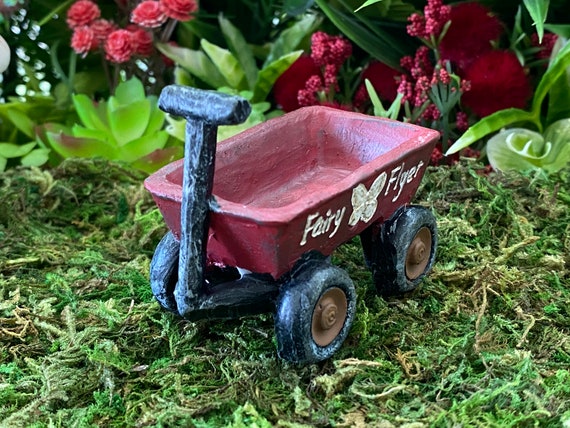This image is a close-up photograph of a small red clay wagon, possibly a delicate decoration or toy. The clay material is evident due to its mostly smooth texture, interrupted by slight imperfections like scratches and dents, likely from the sculptor's fingernails. The edges at the top of the wagon appear lumpy and curved. The wagon bears white text on its side, reading "fairy flyer" with a white butterfly shape between the words. The interior of the wagon is a lighter pink compared to its dark red exterior.

Positioned at a diagonal with the front pointed towards the bottom left, the black handle of the wagon rests against its side, with its black wheels showing brown centers. The wagon sits atop a bed of green moss-like vegetation, perhaps mistaken for grass or weeds. Surrounding the wagon are various succulent plants and what appear to be red carnations, slightly out of focus, with additional green stalks and red berries in the upper left and right corners of the image. The overall scene evokes a garden-like setting, enhancing the whimsical and miniature charm of the wagon.